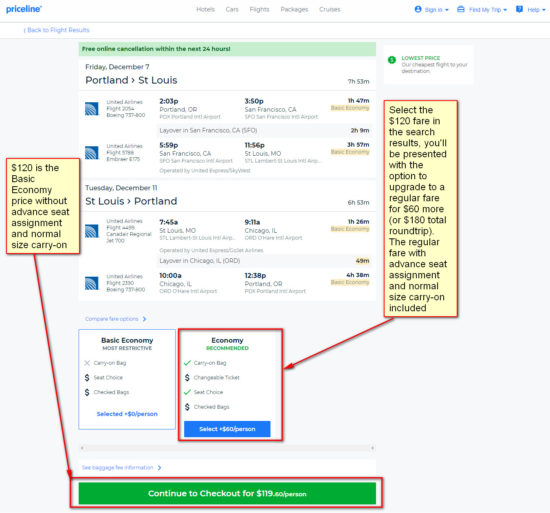In the top left corner, the image displays "Priceline" in blue. Below this, the date "Friday, December 7th" is shown, alongside the text "Portland" with an arrow pointing right towards "St. Louis." To the left, there is a red square with a yellow background containing the text: "$120 – Basic Economy price without advanced seat assignment and normal-size carry-on." A red arrow extends from this box downwards. At the bottom, a green-filled red rectangle reads: "Continue to check out for $119 per person."

On the right side, the image instructs: "Select the $120 fare in the search results. You'll be presented with the option to upgrade to a regular fare for $60 more (or $180 total round trip)." The upgrade includes advanced seat assignment and a normal-size carry-on. A red arrow points down and to the left towards a red square marked "Economy," inside which a blue rectangle displays: "Select at $160 per person."